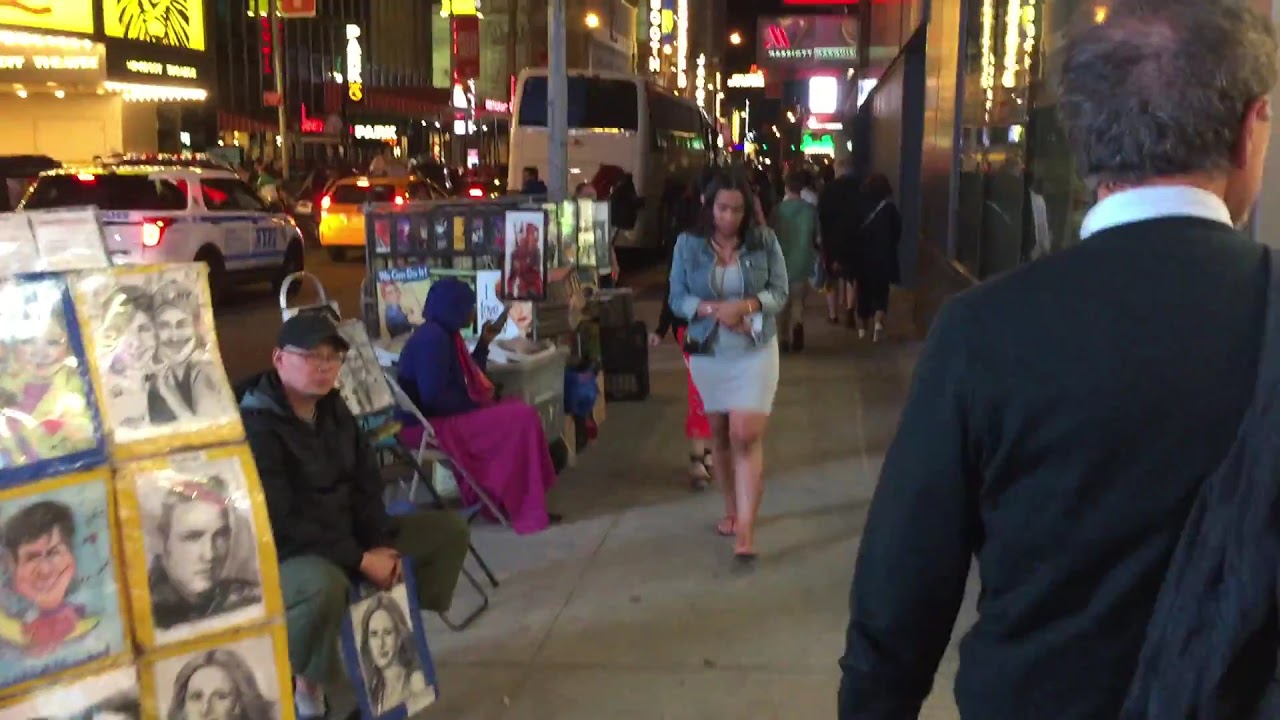In this vibrant nighttime city scene, likely set in downtown New York or a similar bustling metropolis, pedestrians fill the illuminated sidewalks. The foreground features a man in his 50s or 60s, dressed in a black shirt with a white collar, who is pausing to gaze into a store window. Close by, a woman strides confidently forward, dressed in a light blue, tight-fitting miniskirt with a jean jacket and red flip-flops, her brown hair casually falling around her shoulders. She accessorizes with a necklace and a watch on her wrist.

To the left of this woman, art vendors display their work: an array of 8x10 images, including pencil sketches and cartoon-style drawings, set up for sale. One artist, wearing a dark hat and a long-sleeve jacket with green khaki pants, sits by his displayed pieces which feature custom artwork and famous personalities, capturing the interest of passersby. The bustling street extends into the background, with various lit-up signs indicating theaters, restaurants, and a Marriott hotel. The traffic includes a notable taxi van, a police car possibly marked NYPD, and a distinctive white double-decker bus, blending into the busy urban tapestry. The buildings around boast reflective windows, adding to the myriad of lights that animate this lively city landscape.